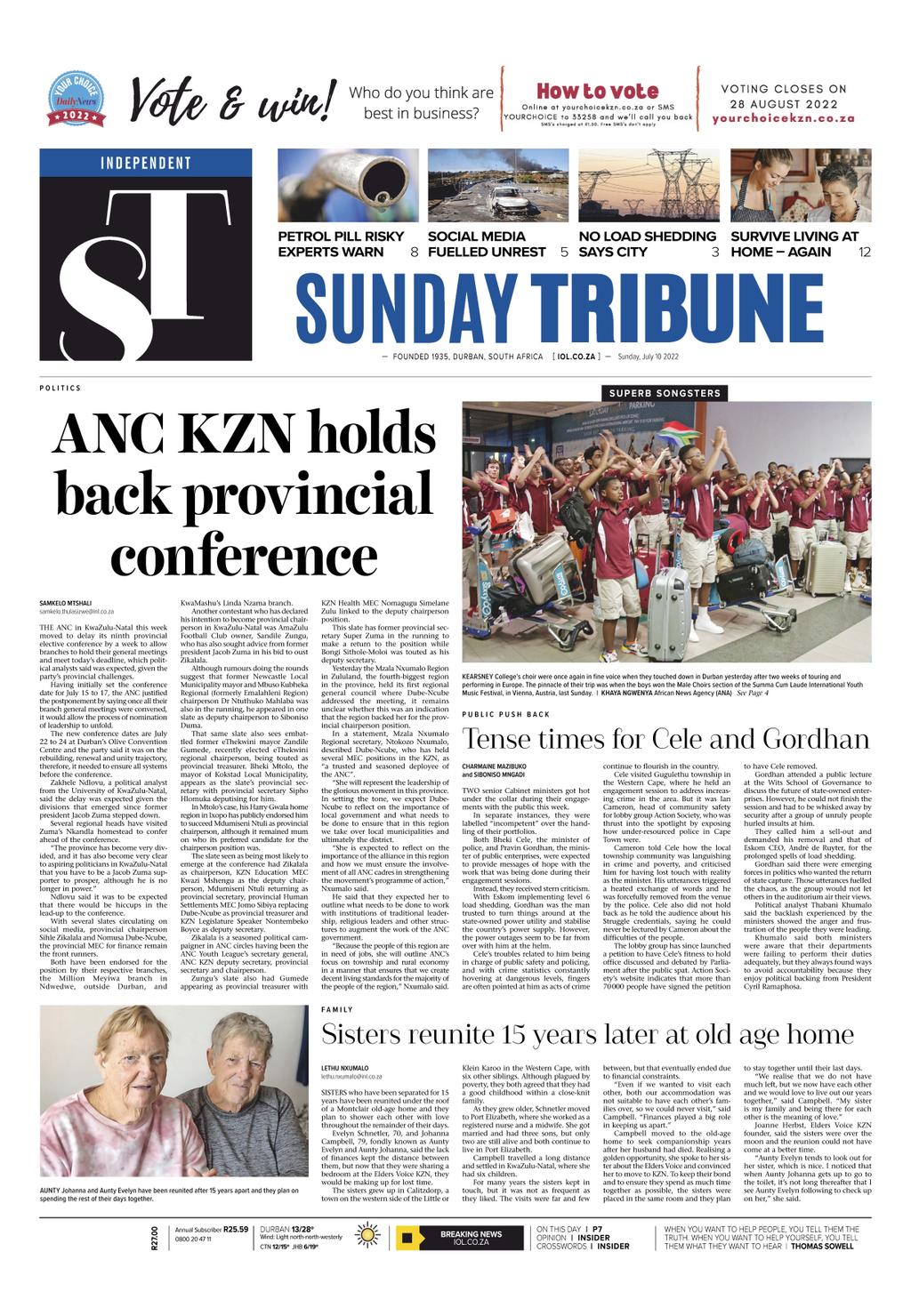**Detailed Descriptive Caption:**

The provided image is a detailed screenshot of the front page of the "Sunday Tribune" newspaper. 

**Header Section:**
- At the very top of the page, the title "Sunday Tribune" is prominently displayed in large, capitalized letters in a medium blue font.
- In the top-left corner, there is a circular logo featuring a red banner which reads "Your Choice Daily News 2022."
- Adjacent to this logo, the phrase "Vote and Win!" is written in black cursive letters.
- Below this, the text "Who Do You Think Are Best in Business?" is followed by "How to Vote," with additional information provided underneath.
- It specifies that voting closes on "28th August 2022" and provides a website for voting details.

**Content Section:**
- Four small images are arranged below:
  1. **Image 1:** Features a pipe and is captioned, "Petrol, Pill, Risky, Experts Warn" with a number eight next to it.
  2. **Image 2:** Shows a burnt car surrounded by debris, captioned, "Social Media Fueled Unrest" with the number five next to the caption.
  3. **Image 3:** Depicts electrical towers with the caption, "No Load Shedding Says City" and marked with the number three.
  4. **Image 4:** Shows an older woman in an apron standing next to a middle-aged woman, with potholders and spices visible on the wall behind them. The caption reads, "Survive Living at Home Again" with the number twelve beside it.

**Newspaper Information:**
- Beneath the images, the "Sunday Tribune" title appears again.
- To the left, there's a square box with a blue bar on top labeled "Independent," against a black background featuring large white letters "S" and "T."

**Publication Details:**
- Below the "Sunday Tribune" title, the text "Founded 1935, Durban, South Africa" is displayed, followed by the volume number and the date "Sunday, July 10, 2022."

**Main Article Section:**
- The main headline reads, "ANC KZN Holds Back Provincial Conference," accompanied by a photo of youths in maroon shirts and khaki shorts at an airport, clapping with their luggage nearby. The group, predominantly composed of black boys with a few white boys present, appears festive.
- A small subtitle, "Public Pushback," is followed by another headline "Tense Times for Cele and Gordon."

**Footer Section:**
- At the bottom of the page, there is a picture of two elderly white women with short hair and noticeable wrinkles, wearing t-shirts. The caption reads, "Sisters Reunite 15 Years Later at Old Age Home."

This front page comprehensively covers various topics, from business voting to social and political issues, providing readers with an array of news and updates.